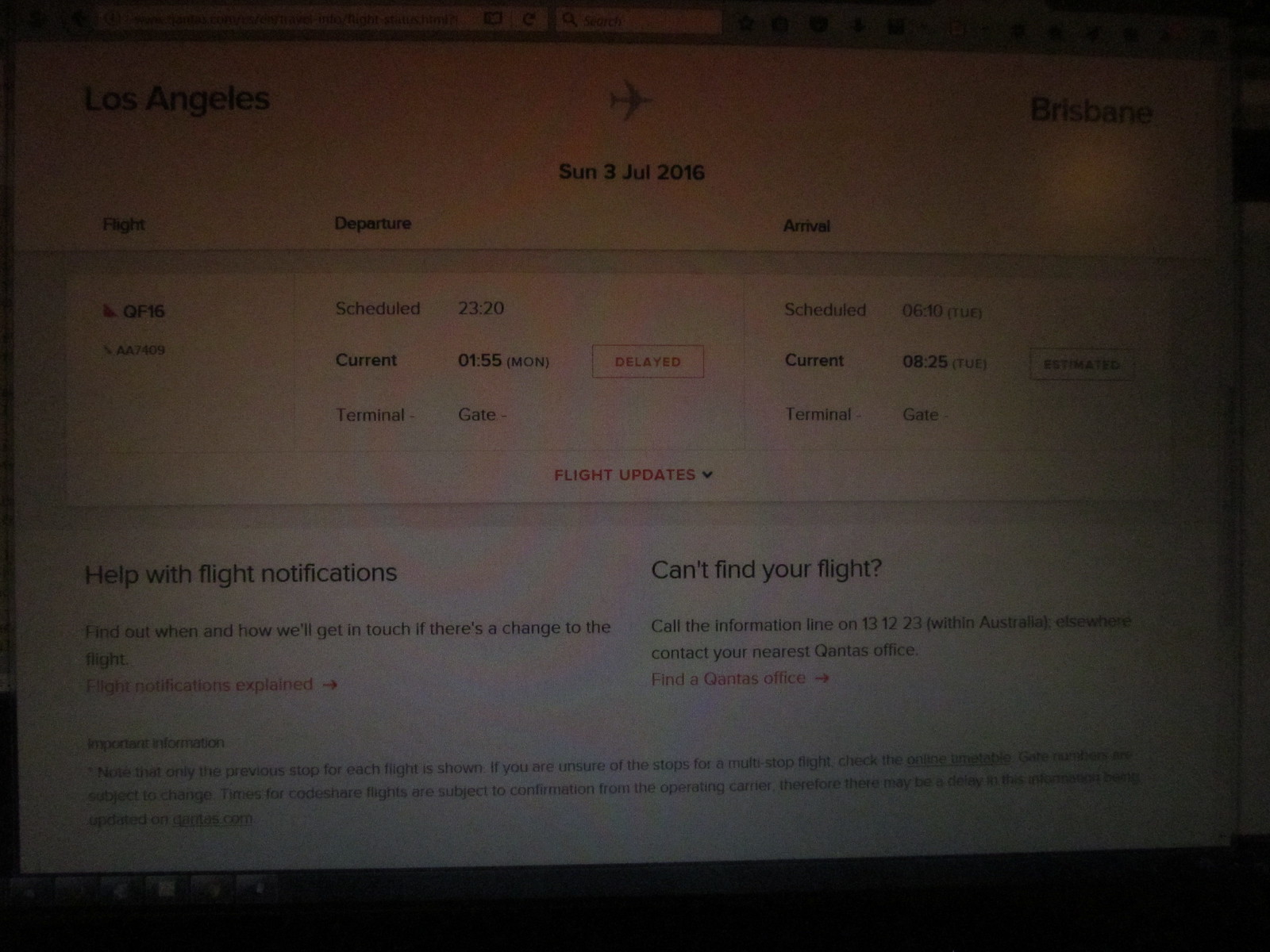This is a dim, grainy photo of a laptop screen displaying a flight itinerary. The screen belongs to a flight from Los Angeles to Brisbane, scheduled to depart on Sunday, July 3rd, 2016, at 23:20 and arrive at 06:10 on Tuesday. An icon of an airplane is visible, indicating the flight path. The flight number is QF16, and the current status includes a delay, with the departure time now shown as 01:55 on Monday and the estimated arrival at 08:25 on Tuesday. The terminal gate information has not been updated. At the bottom of the screen, there are instructions for flight notifications and a helpline number (13 12 23 within Australia) for assistance if the flight details cannot be found, along with a prompt to contact the nearest Qantas office for further help.